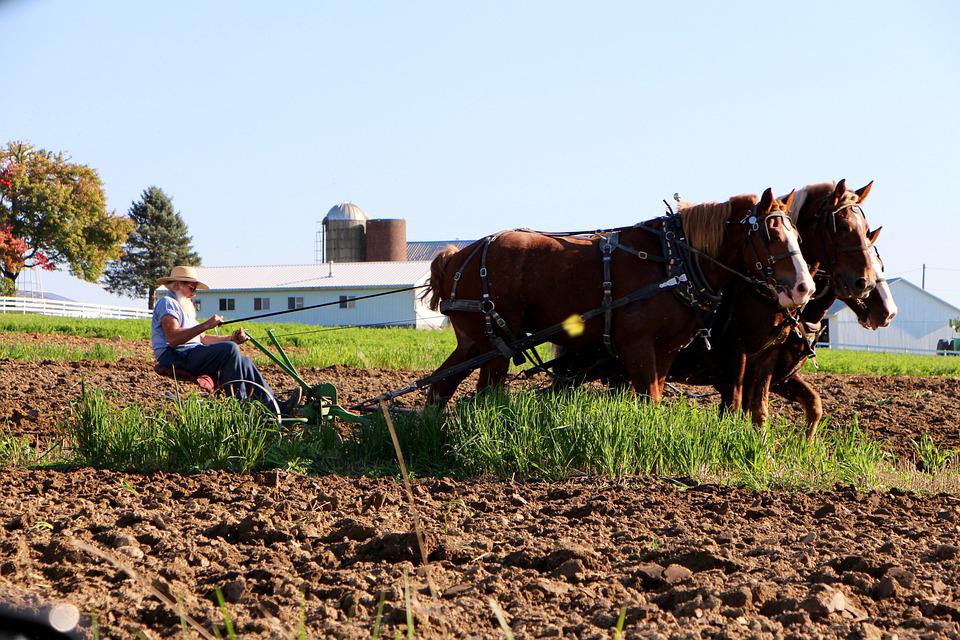In this vivid photograph, a farmer is captured while plowing his field using a small manual plow hitched to three sturdy draft horses. The farmer, adorned with a long white beard, is comfortably seated on the low-riding plow, gripping the reins, and steering the horses as they gently pull ahead. He is dressed in a short-sleeve blue shirt, navy blue pants, and a straw hat that shields his face from the sun. The horses, reminiscent of robust Clydesdales, are brown with light-colored manes and some have white markings on their faces. Their tails are either short or neatly pinned up.

The scene is set in broad daylight under clear blue skies, accentuated by the idyllic countryside setting. The field they are plowing transitions into tall grass, followed by a verdant green lawn. In the background, there are white farm buildings, including a serene barn, a grain silo, and another tower-like structure, framed by sporadic trees. A traditional white picket fence stretches from left to right, adding to the picturesque farm landscape. This image, possibly depicting an Amish farmer from regions like Lancaster, PA or Ohio, showcases not only the diligent labor but also the tranquil and well-maintained environment of rural life.